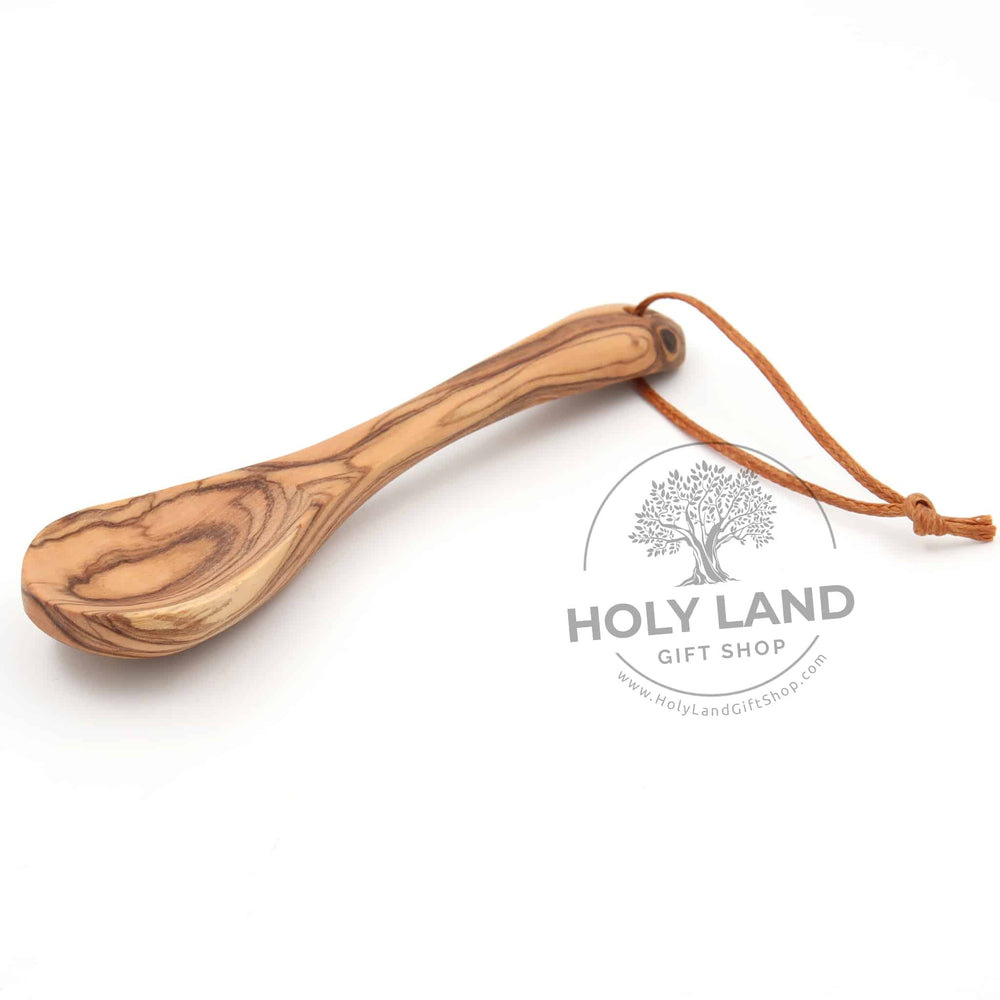The image features a light brown wooden spoon with a prominent grain, resting on a pristine white background. A thick, brownish-orange leather string is threaded through a hole in the handle, possibly for hanging, suggesting a decorative purpose. Below the spoon, a logo in gray depicts a tree outline within a half-circle arc at the top and another half-circle arc at the bottom. Between these arcs, "Hollyland" appears in bold dark letters, while "Gift Shop" is inscribed directly beneath. Underneath the complete circular logo, the website "www.hollylandgiftshop.com" is displayed, indicating that this image serves as an advertisement or business card for the Hollyland Gift Shop.